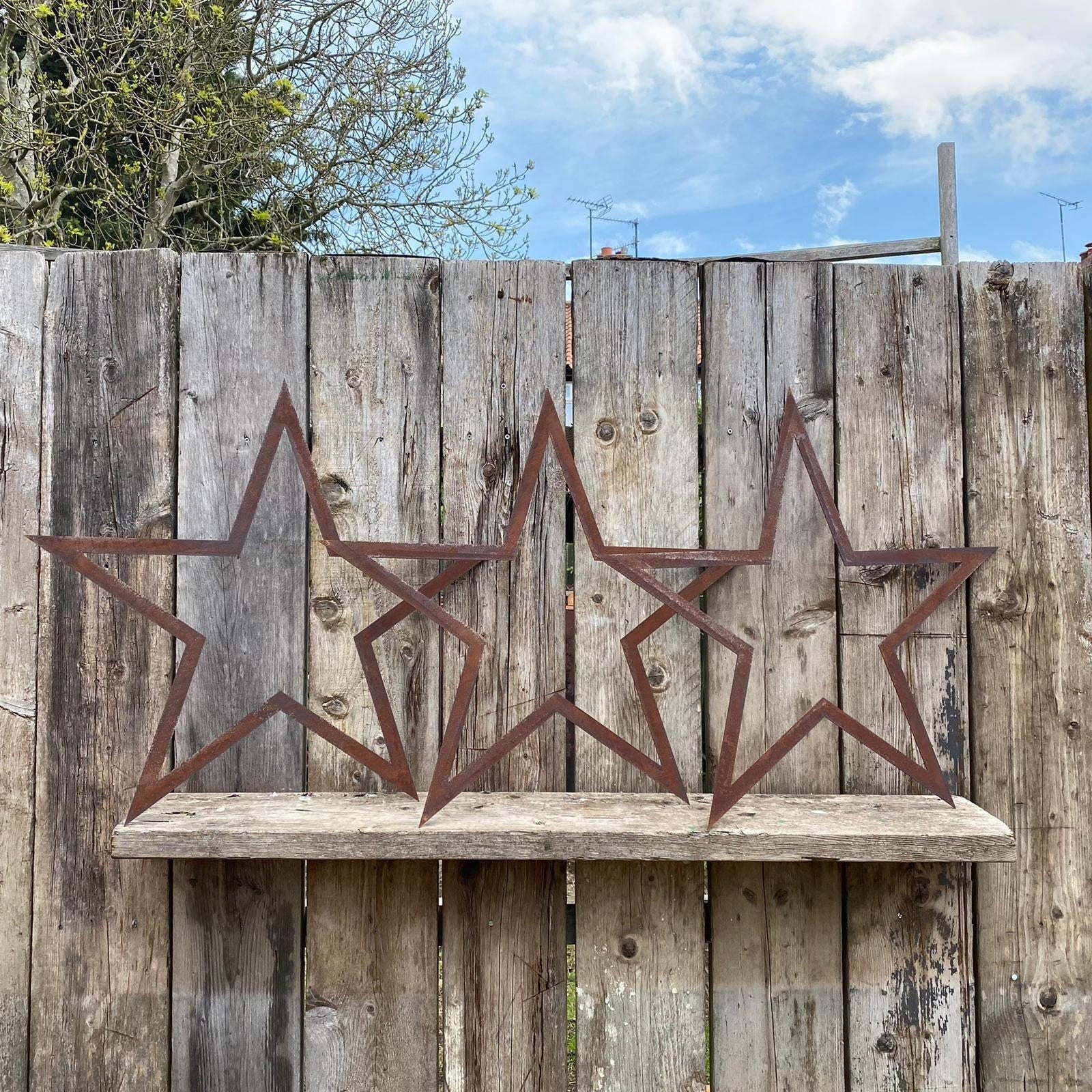The image shows three identical, rusted metal stars with a reddish-brown color, positioned on a weathered wooden shelf that's attached to an old, six-foot tall stockade fence. The fence is made up of variously colored brown planks, some dirtier or lighter than others, with noticeable gaps between some of the planks. The shelf, appearing to be about four feet wide, holds the stars which are aligned next to each other, each with five points. In the background, a vibrant outdoor scene unfolds with a blue sky streaked with wispy white clouds, a few tall green trees peeking over the fence, and a series of telephone poles and other wooden structures visible in the distance. The scene suggests it's the middle of the day.